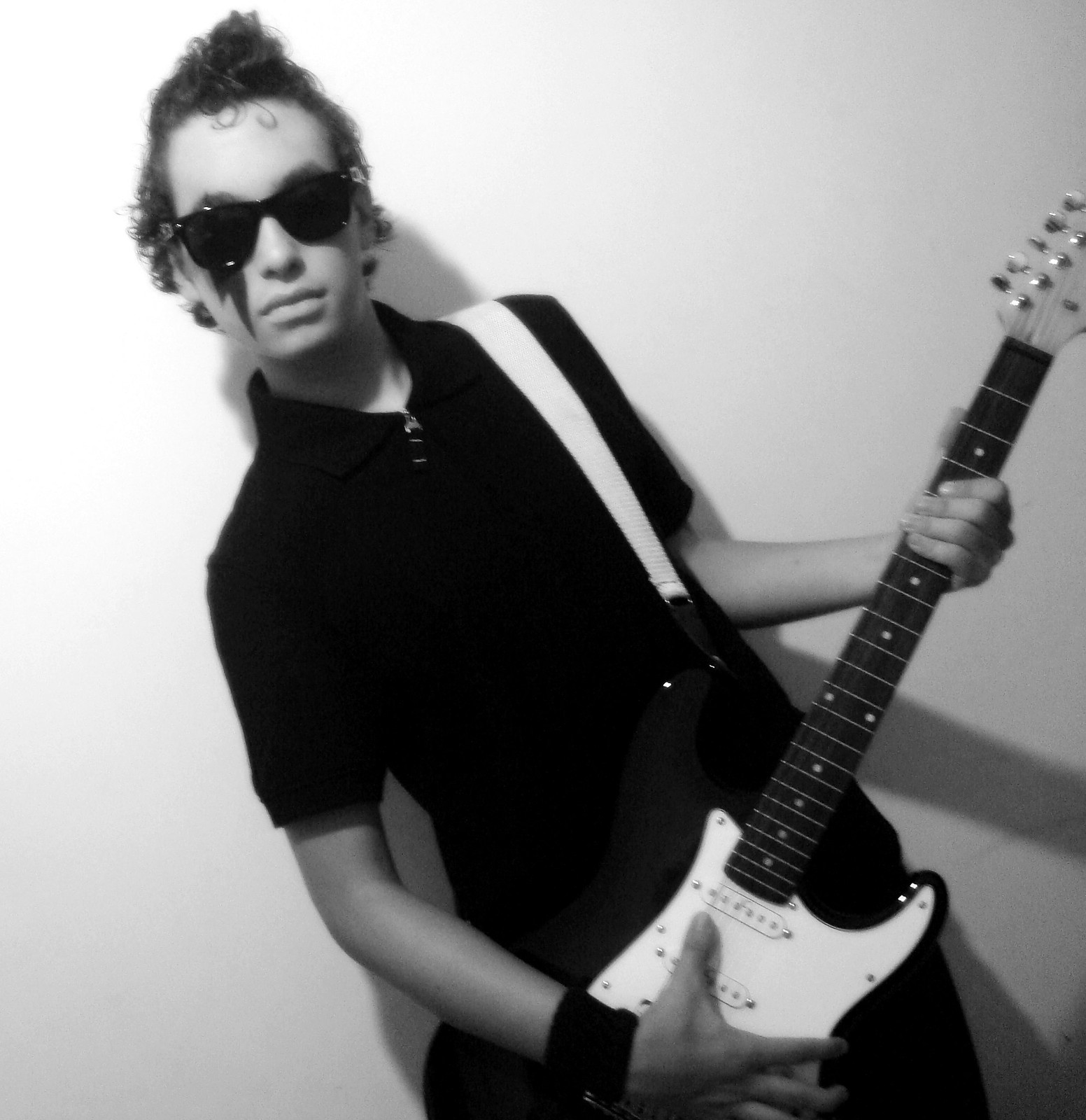In this black-and-white photograph, a young man, possibly in his late teens to early twenties, with light skin and short, curly dark hair, poses against a white wall. He wears black sunglasses and a black wristband on his right wrist. Notably, he has a lightning bolt design or dark face paint on the right side of his face, adding an intriguing element to his look. Dressed in a black t-shirt and black pants, he cradles an electric guitar in his arms, which features a striking contrast of a black body with a white face where he would strum. A white guitar strap is slung over his shoulder. The young man is leaning slightly backward to the left, and his shadow is visible against the wall, enhancing the depth of the image.